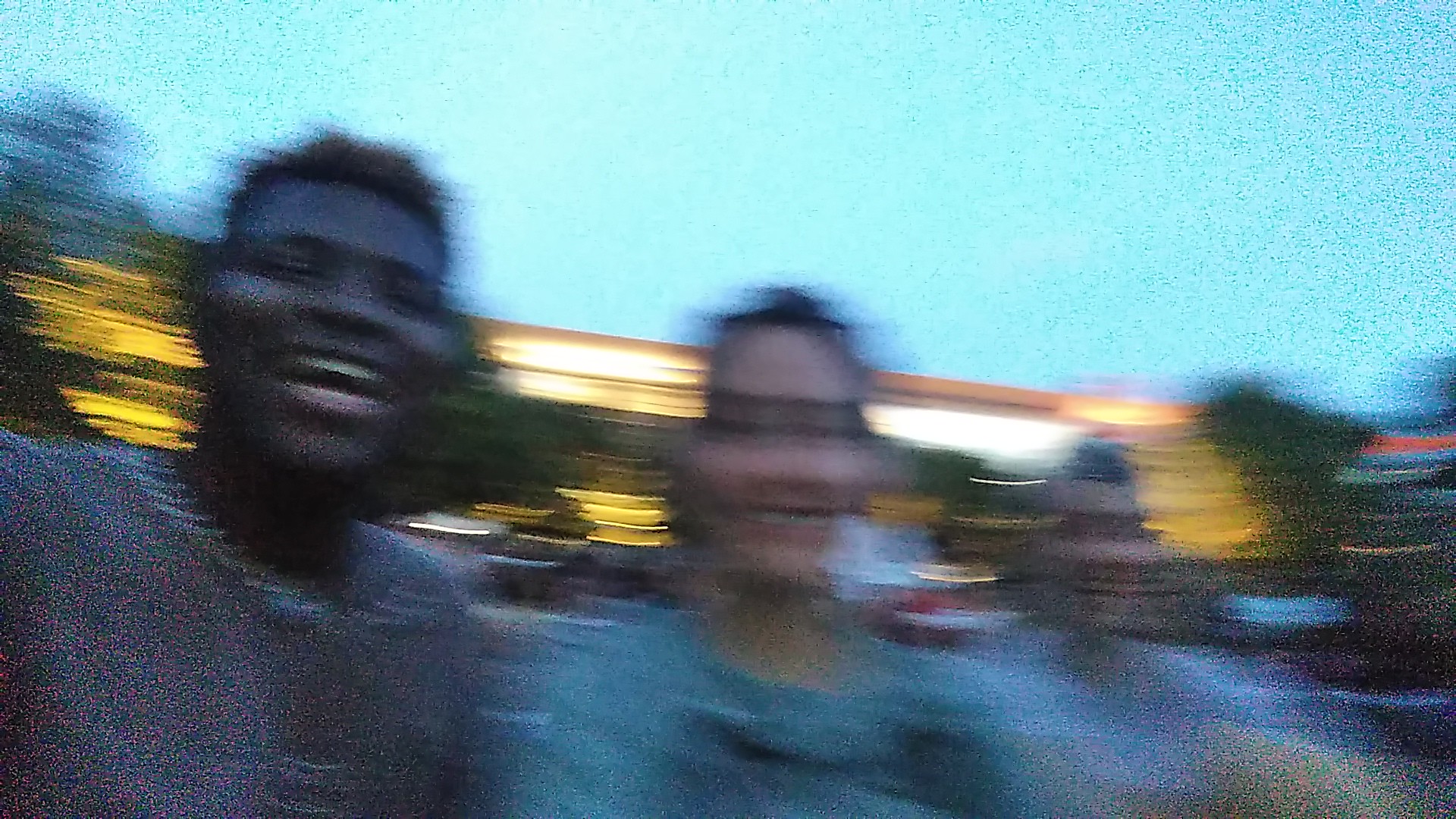In this blurred landscape photo, three people are captured with bright smiles, likely enjoying an amusement park ride as streaks of amber and white lights blur past in the background, suggesting rapid movement. The top half of the image reveals a sky transitioning to evening with a turquoise blue tint. On the left is a dark-skinned man with black hair, prominent cheekbones, and an open, joyful smile, wearing a t-shirt that could be gray. Beside him stands a woman with black hair, high cheekbones, and dark eyes, dressed in a teal or gray jersey-style t-shirt, also smiling warmly. The third person, slightly farther back to the right, is mostly out of focus but adds to the sense of shared excitement. Blurred trees frame the left and right sides of the photo, contributing to the lively, dynamic scene.